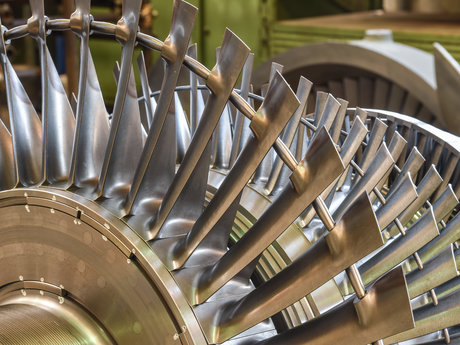The image showcases three intricately designed steel objects, each formulated into a circular pattern resembling wheels or gears. The centerpiece of each object is solid, from which elongated, fan-like structures or pillars protrude radially, giving them a strikingly intricate and industrial appearance. These metallic objects are metallic and reflective, capturing and mirroring the surrounding light. They are lined up sequentially in the foreground, with a close-up, panned-in perspective emphasizing their detailed craftsmanship.

In the background, the scene suggests an outdoor setting, with visible greenery, grass, and some steps, hinting that these objects might be part of an outdoor exhibit, possibly in a park or an open-air foyer of a building. However, another interpretation suggests they could be part of an indoor display, given the reflective quality of the light, and the presence of a light green section that might be a wall or cabinet. Regardless of the exact setting, the image captures the complexity and beauty of these industrial-looking steel structures.